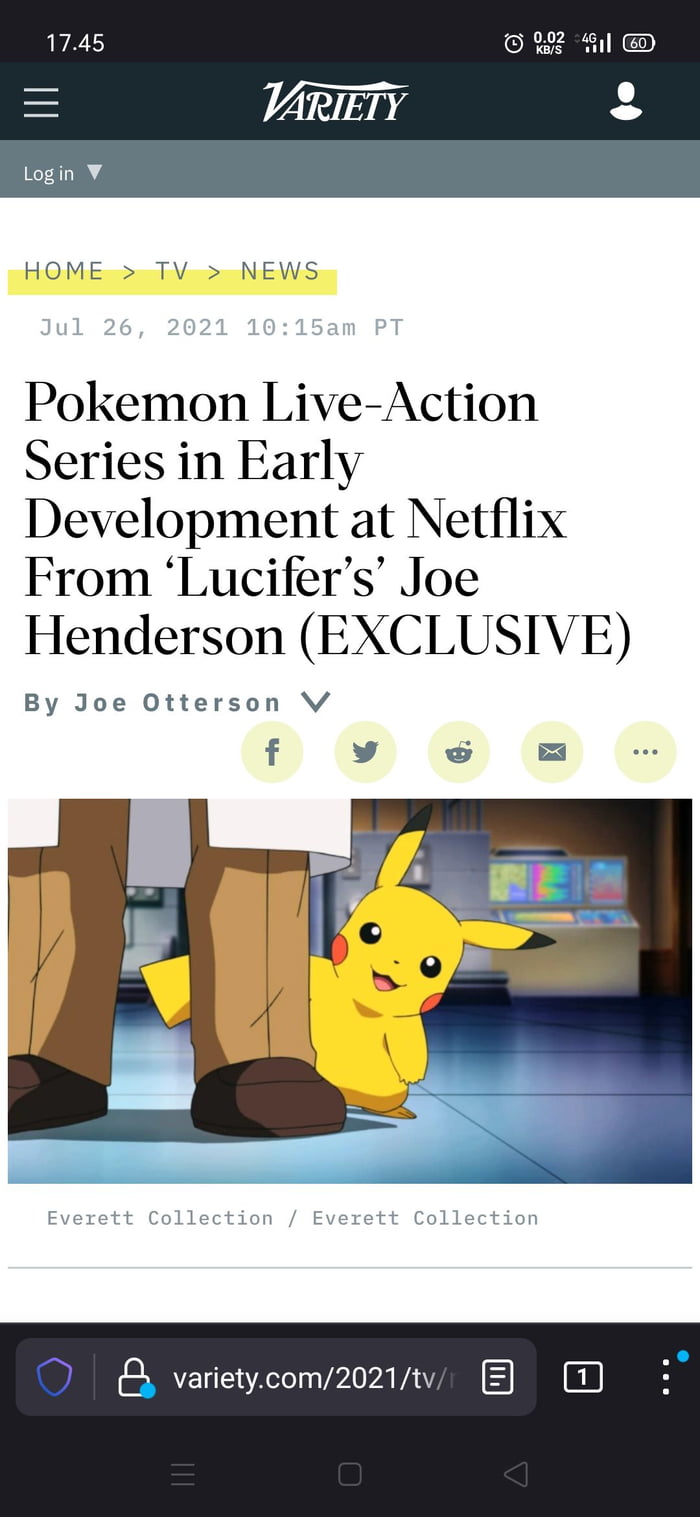This screenshot, captured on a smartphone, highlights a post from Variety. The main content of the post announces a "Pokémon live-action series in early development at Netflix," exclusively reported by Joe Henderson, known for his work on 'Lucifer.' 

In the upper left-hand corner of the screenshot, the time is displayed as 17:45 in white text. The upper right-hand corner features several status icons, including battery percentage, Wi-Fi signal strength, and additional indicators, all set against a dark gray background. Below this, there is a slightly larger gray bar with 'Variety' centered in white text. To the left of this text are three horizontal bars, presumably a menu icon, and to the right is an icon resembling a contact book or user profile.

Further down, a lighter gray bar features a 'Login' option on the left-hand side, indicated by a dropdown arrow. Highlighted in yellow within the main article navigation are the categories: 'Home,' 'TV,' and 'News.' The article itself, authored by Joe Otterson, begins below these navigation options, with the title emphasizing the development of the Pokémon live-action series. Accompanying the article text is an image related to Pokémon, adding visual context to the announcement.